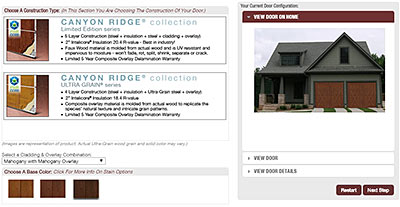**Caption:**

The image showcases various garage door options against a white background, specifically from the Canyon Ridge Collection. At the top left, it reads "Choose a construction type," but the text is difficult to decipher due to the small image size. Below that, a prominent rectangular blue box displays "Canyon Ridge Collection," highlighting the Limited Edition Series and its distinguishing features. To the immediate left of this box is a dark brown garage door representing the Limited Edition Series.

Below this first section, text introduces the "Canyon Ridge Collection Ultra-Grain Series," accompanied by another set of highlights. Adjacent to this text, there is a lighter brown garage door which is solid in color.

Further down, under the heading "Select," there's a dropdown menu displaying an option for "Mahogany with Mahogany Overlay." Following is a section instructing users to "Choose a base color" and to click for more information on finish options. This section includes three color swatches: a light brown on the left, a solid brown in the middle, and a dark brown on the right.

To the right of this selection, a bordered area invites customers to "View Door on Home," featuring a stock image of a house with a garage door. Below this visual, buttons provide options to "View Door Details" and to "Restart Next Step," each accompanied by brown buttons for easy navigation.